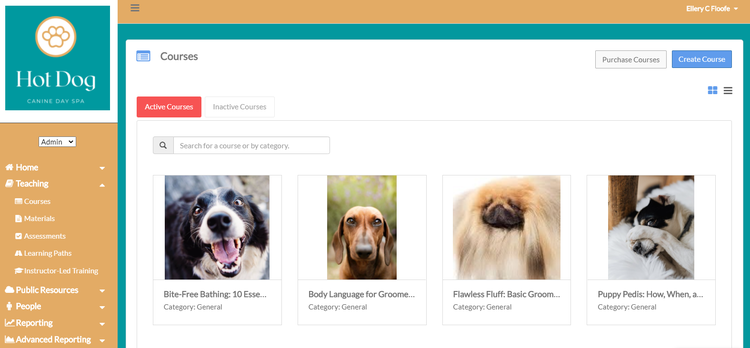Caption:
An image from the "Hot Dog" website showcases a vibrant, canine-themed interface. In the top-left corner, a brown-colored dog's paw illustration is prominently featured against a white background. The site name, "Hot Dog," is displayed in a green box with the paw at the center. Below, the banner reads "Canine Day Spa."

On the left side, a navigation menu lists the following options:

- Admin
- Home
- Teaching Courses
- Materials
- Assessments
- Learning Paths
- Instructor-Led Training

Under a cloud icon labeled "Public Resources," there is a person icon for "People" and a line graph icon for "Reporting." At the bottom, another icon labeled "Advanced Reporting" is present, each featuring drop-down menus.

The top of the page features a "Courses" section with categories for "Active Courses" and "Inactive Courses." Highlighted active courses include:
- Bite-Free Bathing
- 10 Essentials
- Body Language for Groomers
- Flawless Fluff Basic Grooming
- Puppy Pals

Additional options for "Create Courses" and "Purchase Courses" are visible. The section also showcases four images of dogs, enhancing the site's engaging and pet-friendly atmosphere.